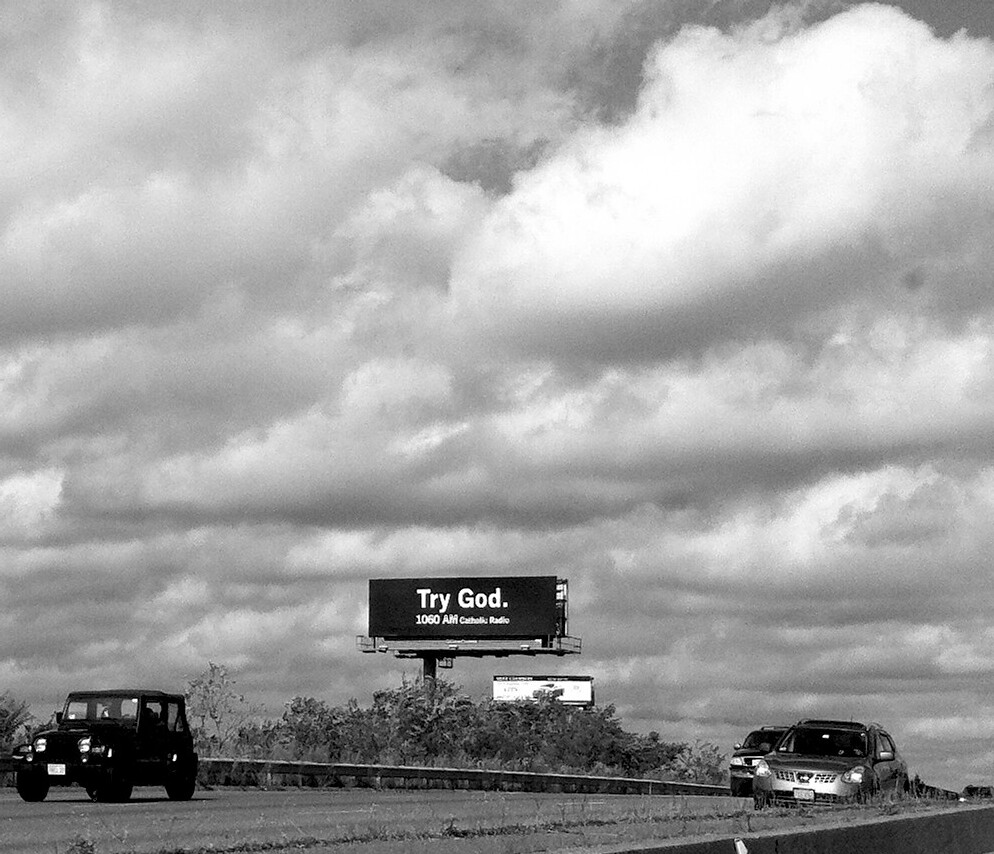In this evocative black-and-white photograph, a four-lane highway stretches across the frame, drawing the viewer's eye towards the horizon and a landscape dominated by a foreboding, overcast sky. The oppressive clouds seem to rest on an invisible barrier, intensifying the scene's moody atmosphere. On the highway, three vehicles are captured heading towards the camera: a Jeep, a truck, and an SUV parked on the median. To the right, the road's edge is visible in the lower-right corner, marked by trees and a guardrail. A striking black rectangular billboard stands prominently on the median, bearing the bold white text, "Try God," followed by the smaller inscription, "1060 AM Catholic Radio." Another, illegible billboard appears far in the background, subtly enhancing the depth of the scene. The raw drama of the looming sky contrasts with the grounded activity on the roadway, creating a powerful and layered visual narrative.